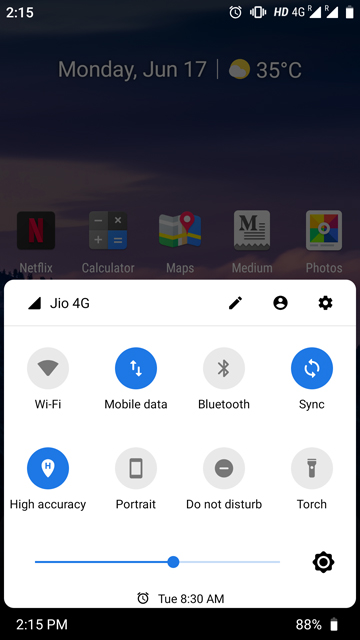The image displays the screen of a user's smartphone. At the very top-left corner, the time is shown as 2:15 in white text. To the right of the time display, several status icons indicate the phone's status: the battery is nearly full at 88%, signal strength is full for 4G, and an alarm is set. Directly underneath, white text reads "Monday, June 17," alongside a temperature of 35 degrees Celsius. An orange-yellow ball symbol, either representing a full moon with a small cloud in front of it or a sun, is also visible.

Below this status information, several apps are visible on the user's home screen, including Netflix, Calculator, Maps, Medium, and Photos. An open tab at the center of the screen displays a white box featuring a settings icon in the bottom right corner, an edit button, and a contacts icon in the top right.

Within this white box, two horizontal rows of options are displayed:
- The top row includes Wi-Fi, Mobile Data, Bluetooth, and Sync.
- The bottom row consists of High Accuracy, Portrait, Do Not Disturb, and Torch.

Among these options, Mobile Data, Sync, and High Accuracy are highlighted in blue, indicating they are active. The volume slider is set at the 50% mark.

Towards the bottom section of the screen, an alarm is shown to be set for 8:30 a.m. on Tuesday. Finally, at the very bottom left corner, the display again shows the time as 2:15 p.m., with the battery life indicated at exactly 88%.